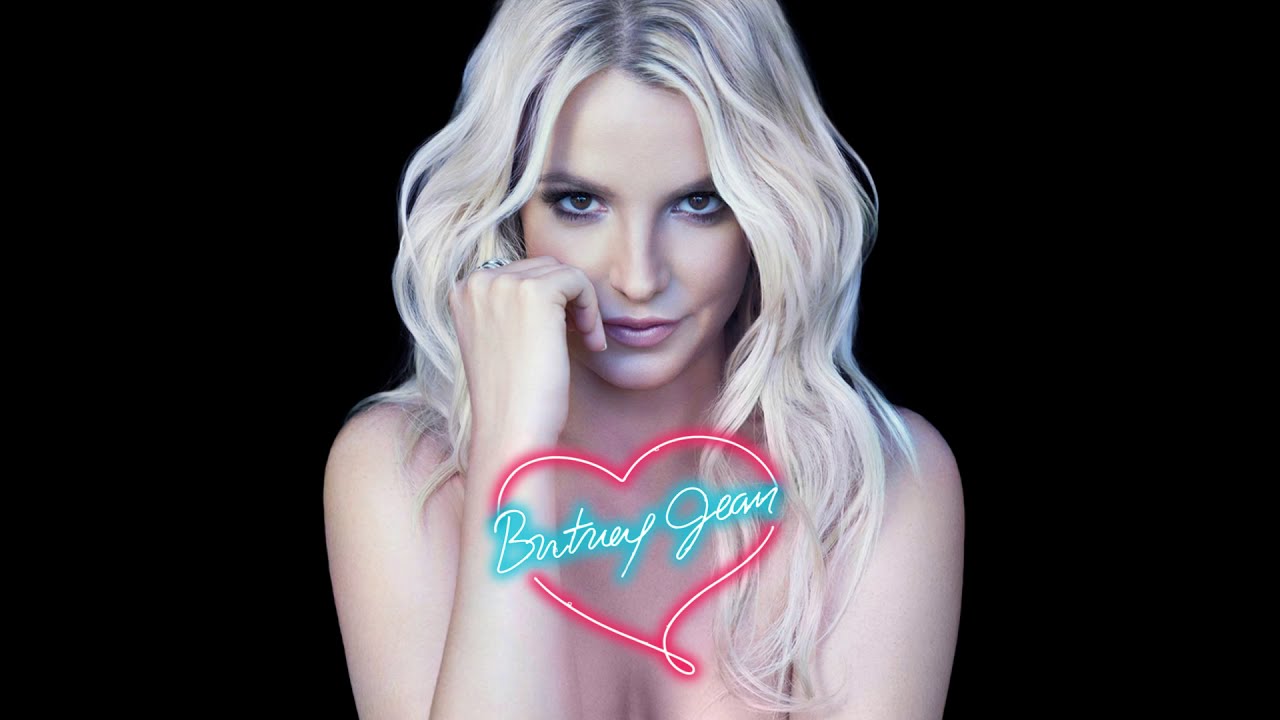The image features a digitally retouched photograph of a young Britney Spears, centered against a pitch-black background. Britney is depicted from her head and shoulders down to nearly her elbows, with her pose revealing pale white skin and long blonde hair cascading over her shoulders. She appears topless, though her positioning and hair obscure any possible clothing details. Her right arm is bent, with her hand raised near her face, and she wears a ring on her third finger. She gazes straight ahead with a sultry, seductive expression. In front of her chest, a neon graphic spells out "Britney Jean" in blue cursive, surrounded by a red neon heart outline, giving the entire composition a vibrant, almost sticker-like appearance.